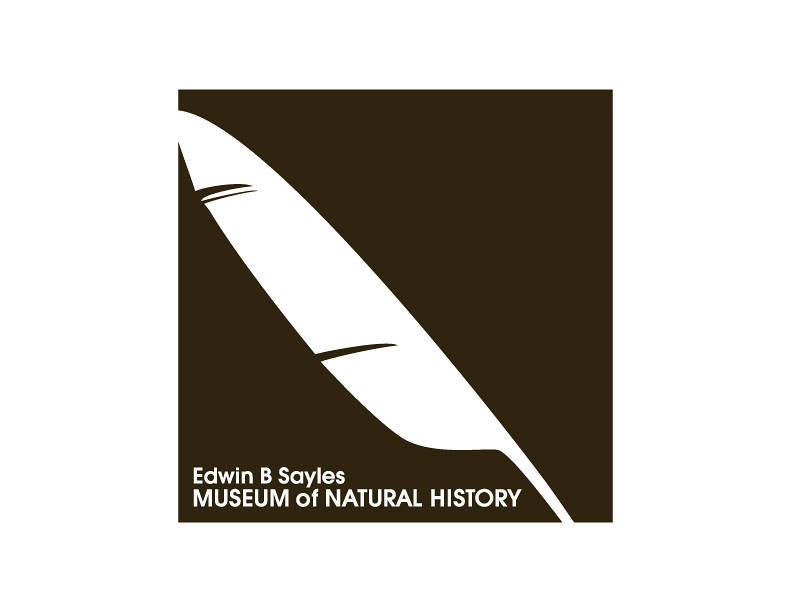The image is a small, square advertisement with a black background. Dominating the frame is a white feather that stretches diagonally from the top left to the bottom right. The feather is mostly solid white but features a few lines of separation that give it a more realistic texture. In the bottom left corner, the text reads "Edwin B. Sayles" in small white letters, with "Museum of Natural History" in larger, capitalized white letters beneath it. The overall design suggests a promotional piece for the museum, emphasizing the feather as the central motif.